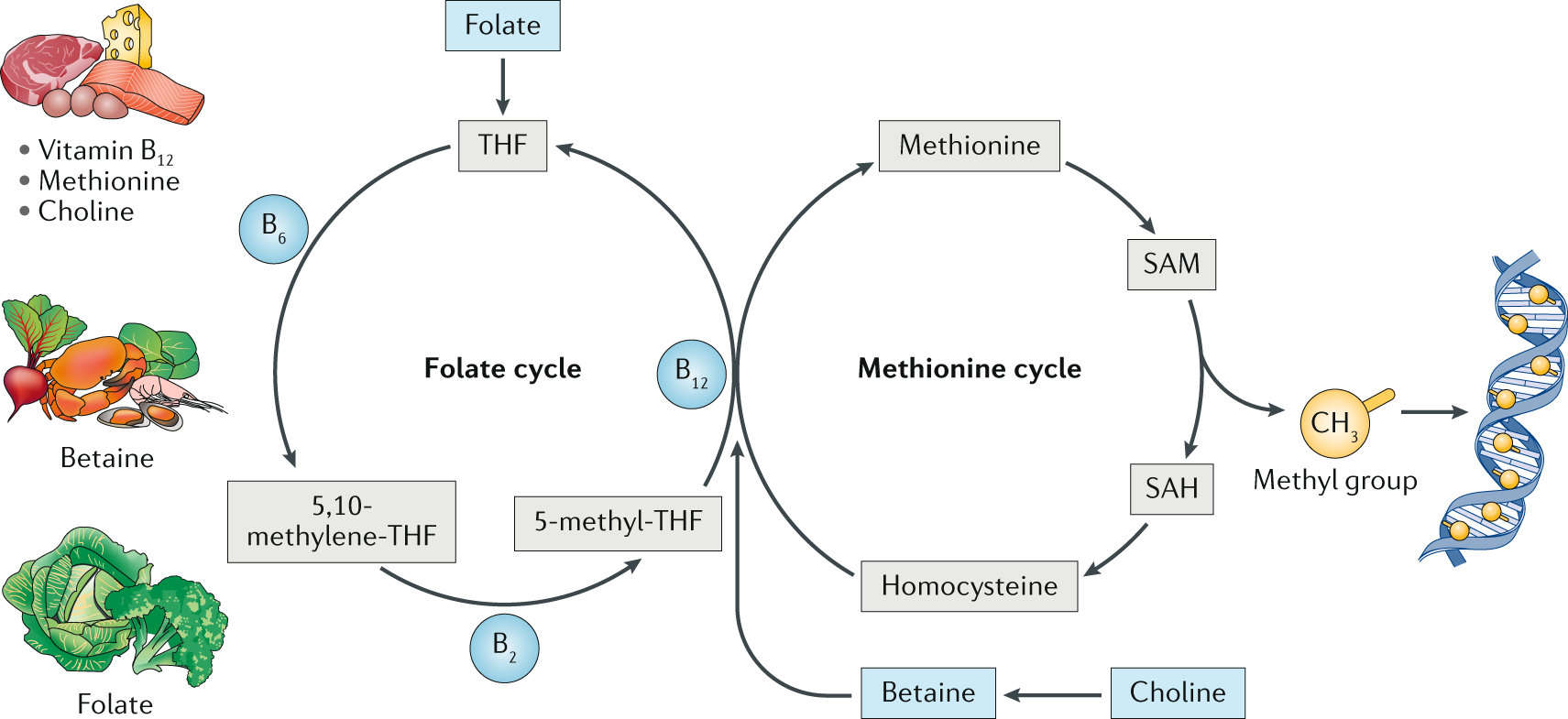This image is a detailed scientific diagram illustrating the folate cycle and methionine cycle. At the center, two interconnected circles—one labeled "Folate Cycle" and the other "Methionine Cycle"—feature arrows indicating the cyclical flow through various chemical compounds such as B2, B6, B12, methionine, homocysteine, choline, SAM (S-adenosylmethionine), and SAH (S-adenosylhomocysteine). To the left of the cycles, three distinct food groups are shown. The first group, associated with vitamin B12, methionine, and choline, includes representations of steak, eggs, salmon, and cheese. The second group, linked to betaine, features crab, beets, leafy greens, shrimp, and oysters. The third group, related to folate, displays broccoli and cabbage. This comprehensive chart connects nutrient sources to their biological roles, possibly serving as an educational tool in a biology or medical setting.